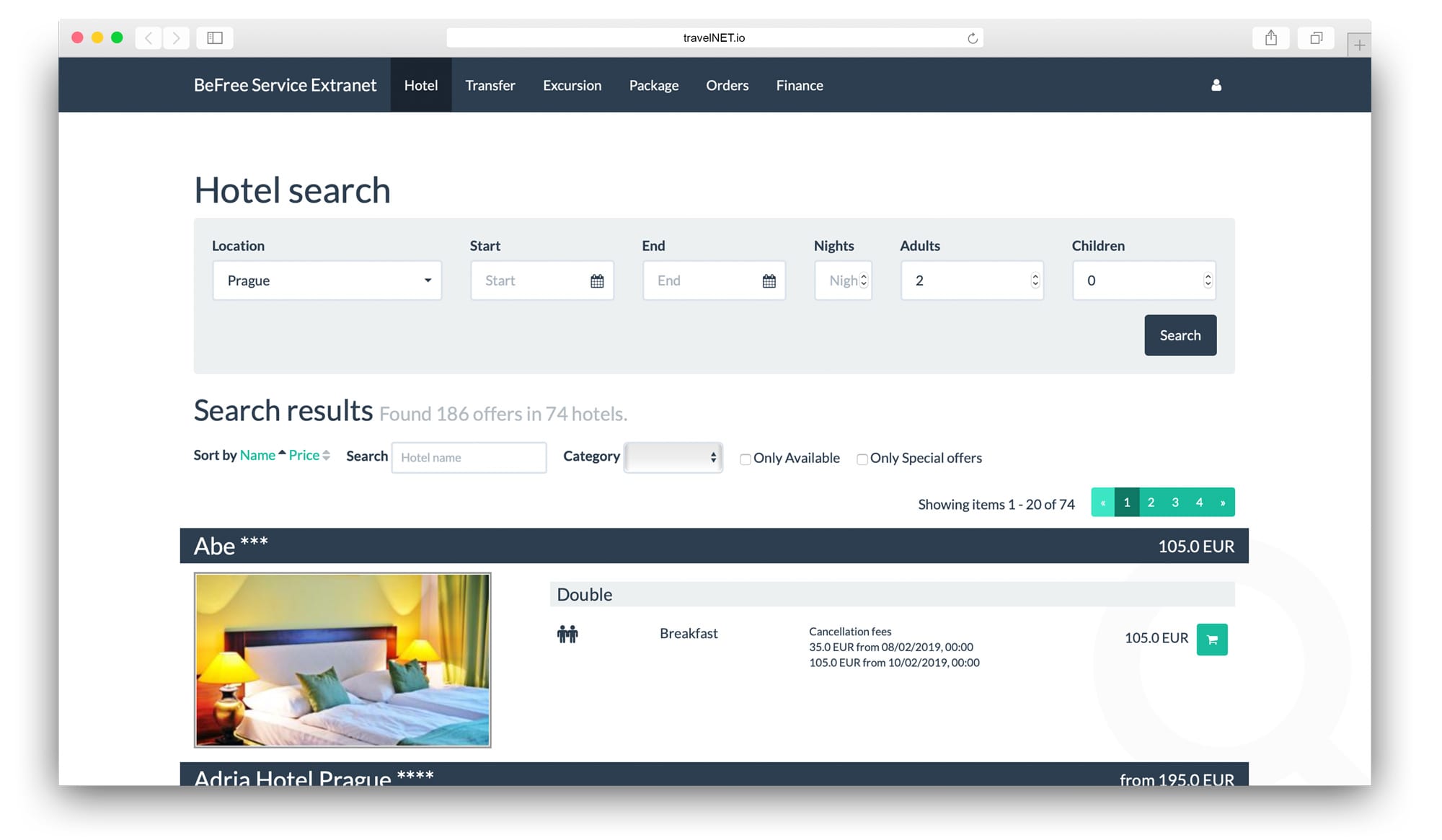### Detailed Caption for Hotel Search Website Screenshot

The screenshot displays a hotel search website page against a white background. At the very top, there is a navigation bar featuring three colored circles (red, yellow, green) on the left, followed by a back arrow, a forward arrow, and a page icon. In the center, there appears to be a search box containing some text, alongside an undo button. To the right side of this navigation bar, there is a shopping bag icon and a minimize icon.

Directly below the navigation bar, a blue banner spans across the screen with white text stating "Be Free Service Extranet Hotel," which is highlighted. This banner also includes options for "Transfer," "Excursion," "Package Orders," and "Finance," with a profile icon situated on the far right.

Beneath the blue banner, large dark blue text reads "Hotel Search." A gray input box is displayed indicating "Location: Prague," with the fields "Start," "End," "Nights," "Adults" (defaulted to two), and "Children" (defaulted to zero) available as dropdown boxes. To the right of these options, a dark blue button with white text prompts users to "Search."

Following the search section, detailed search results are presented, revealing a total of 186 offers spanning 74 hotels. Users can sort these results by "Name" or "Price," both of which are indicated as green hyperlinks. Additionally, there are checkboxes available to filter results for "Only Available" and "Only Special Offers." A line below specifies that the interface is showing offers 1 through 20 out of 74.

An example of one search result is highlighted, beginning with the label "Abe" next to an image of a hotel bed. Additional details for this offer include "Double Breakfast," "Cancellation Fees," and a price listed at "105 euros."